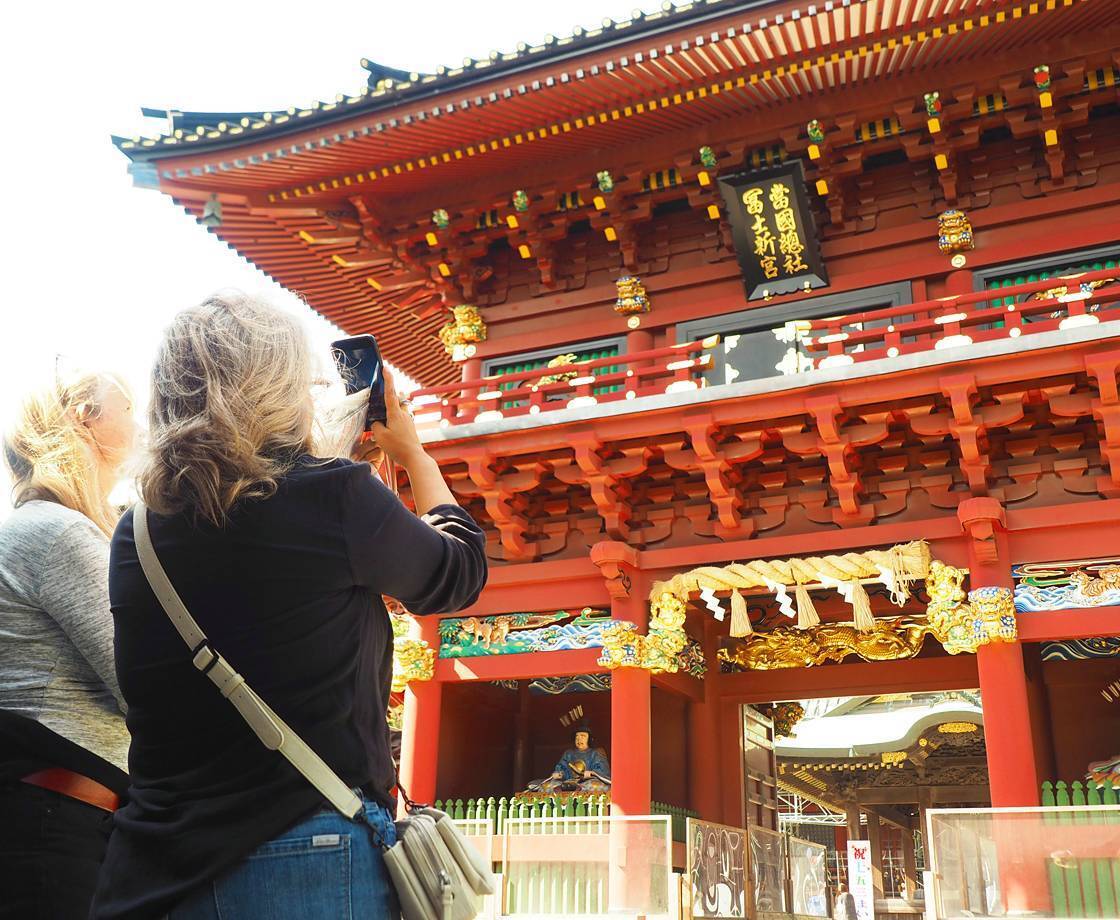The image depicts an expansive, traditional Asian structure, likely a Chinese or Japanese house, characterized by a red facade with black and gold accents. The building features a pagoda-style roof with square but upward-tilting eaves. Above the entrance, there is a black rectangular plaque with gold Asian characters. In the foreground, two blonde women, appearing to be tourists, stand near the building. One woman, dressed in a light gray shirt and black pants, is observing the surroundings, while the other, with her hair pulled back and dressed in a black shirt and denim jeans, is capturing the scene on her smartphone, a white purse strapped across her back. The setting appears to be an outdoor daylight scene, lending to the authenticity and cultural significance of the location.